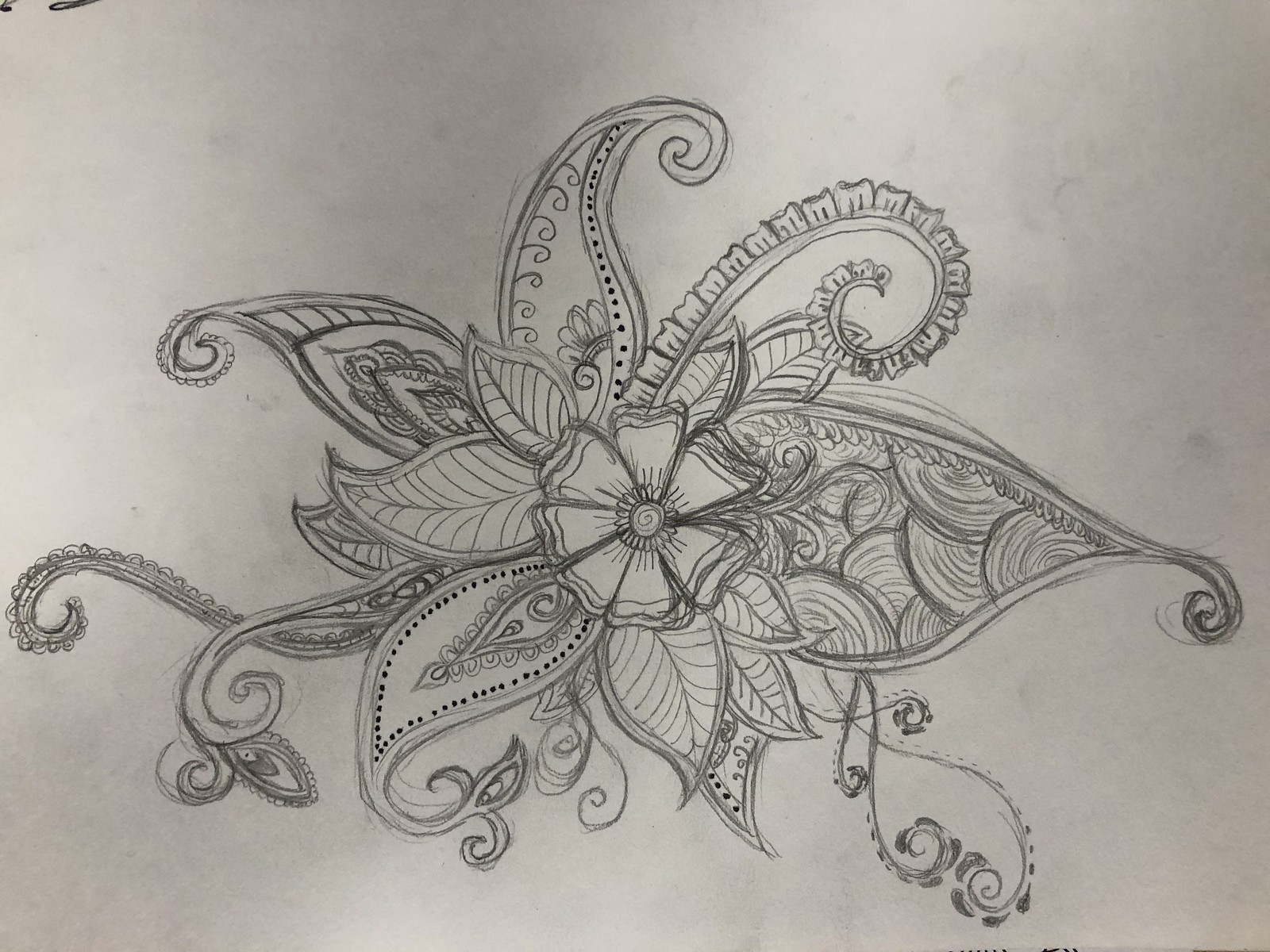The image is a detailed pencil drawing on a piece of dull, off-white paper. At the center of the drawing is a flower with seven petals, resembling a daisy. Radiating out from this central flower are numerous ornate leaves, each with unique, intricate designs. Some leaves feature swirling or scroll patterns, while others have detailed veins or resemble teardrop shapes with circular designs within them. One particularly notable leaf on the right side of the flower features a circular pattern, ending in a scroll design. Other leaves extend outwards, winding around like octopus arms, and some exhibit an almost fleur-de-lis motif with dots. The overall composition is highly decorative, with the leaves and their varied patterns spiraling around the central flower, creating an elaborate and artistic effect.